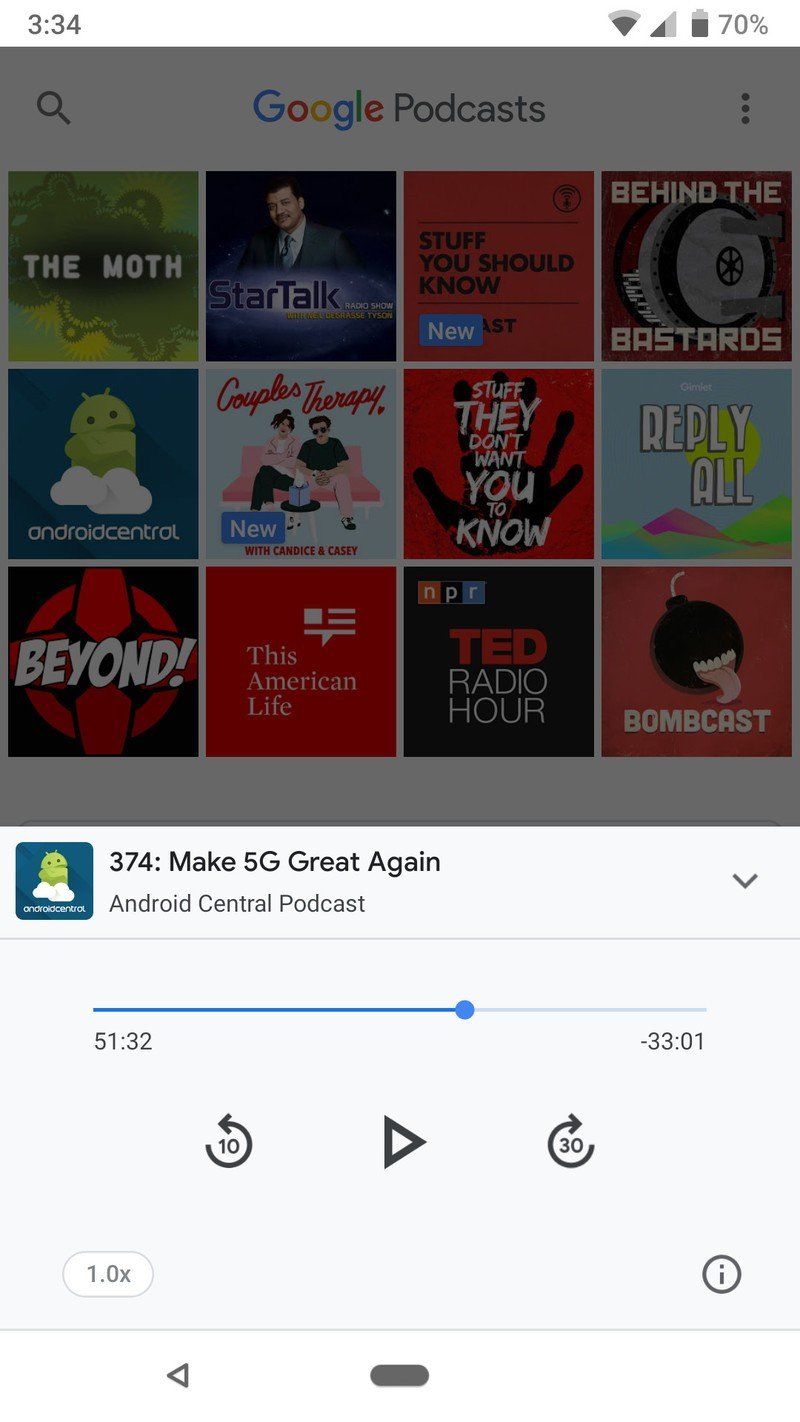The screenshot captures a mobile webpage interface with various elements and sections. 

At the top left corner, there are status icons including time "3:34," Wi-Fi signal strength, phone service signal strength, and a battery icon indicating "70%." Below this is a white background with a partly obscured gray dialog box.

On the upper left side of the image, there's a black magnifying glass icon for search. Next to it, the title "Google Podcasts" appears with the Google logo in its signature colors (blue, red, yellow, blue, green, red) followed by the word "Podcasts" in black. To the right, three vertical dots symbolize a menu.

The main section of the screen has three rows, each featuring four podcast icons:

1. **Top Row:**
   - **The Moth**: Green background with white text.
   - **StarTalk**: Image of a black man in a suit.
   - **Stuff You Should Know**: Red background with black text and a blue "New" banner in the bottom left.
   - **Behind the Bastards**: Image of a gray vault with white text at the top ("Behind Me") and bottom ("Bastards").

2. **Middle Row:**
   - **Android Central**: Blue box with a green Android symbol. Below, in white it says "Android Central."
   - **Couple Therapy**: Blue background featuring a woman in a pink shirt and a man in sunglasses with a black T-shirt. Pink text at the top reads "Couple Therapy."
   - **Stuff They Don't Want You to Know**: Red background with a black handprint and white text.
   - **Reply All**: Black background with a cartoony sun, rainbow-colored mountains, and white text.

3. **Bottom Row:**
   - **Beyond**: Black background with a red symbol and white text.
   - **This American Life**: Red text on a black background.
   - **TED Radio Hour**: Red text "TED" and white "Radio Hour" on a black background.
   - **Bombcast**: Red box with a black bomb image. White text reads "Bombcast."

At the bottom of the screen is a white box with various detailed podcast information:
   - At the top left, a tilish blue rectangle with a green Android symbol.
   - To the right, black text reads "374, Make 5G Great Again."
   - Below, the title "Android Central Podcast" appears.
   - A downward-pointing arrow is to the right.

A blue progress bar stretches across, showing a halfway point identified by a blue circle. Below the bar, "51:32" is on the left, possibly indicating the time elapsed, while "33:01-" is on the right. Navigation icons include a left-pointing arrow with "10" inside, a black play symbol, and another right-pointing arrow with "30" inside.

At the very bottom, a white bar with "1.0x" in gray is seen. To its right sits a black circle containing a lowercase "i."

This detailed caption aims to provide a vivid and exact description of the screenshot, highlighting each element and its corresponding details.